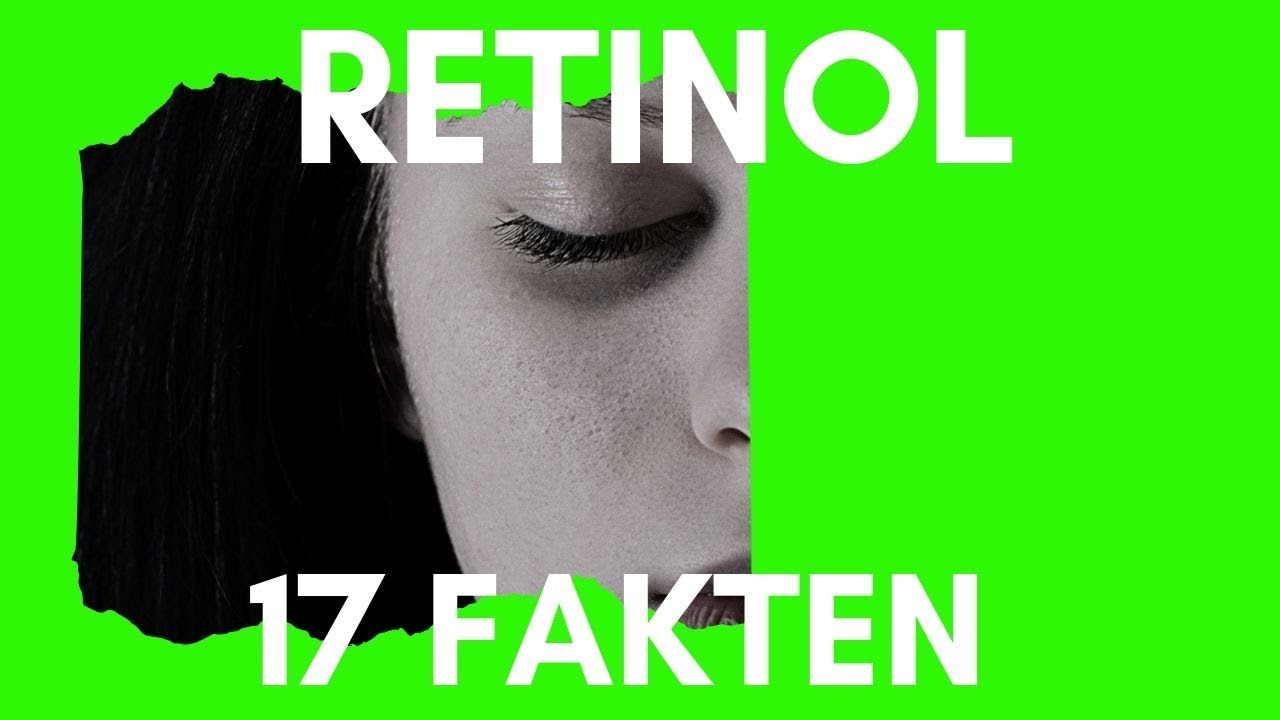The image features a rectangular, magazine-like ad dominated by a bright, almost neon green background. On the left side of the ad, there is a close-up, black-and-white photo of the right side of a young woman’s face, highlighting her eyebrow, eye, half of her nose, lips, and her right cheek. A small part of her hair is also visible against a dark black background. The focal point seems to be on the texture of her skin, particularly her pores. The ad prominently displays text in large white block letters, with "retinol" at the top and "17 Fakten" at the bottom, suggesting a German context for the product or message.